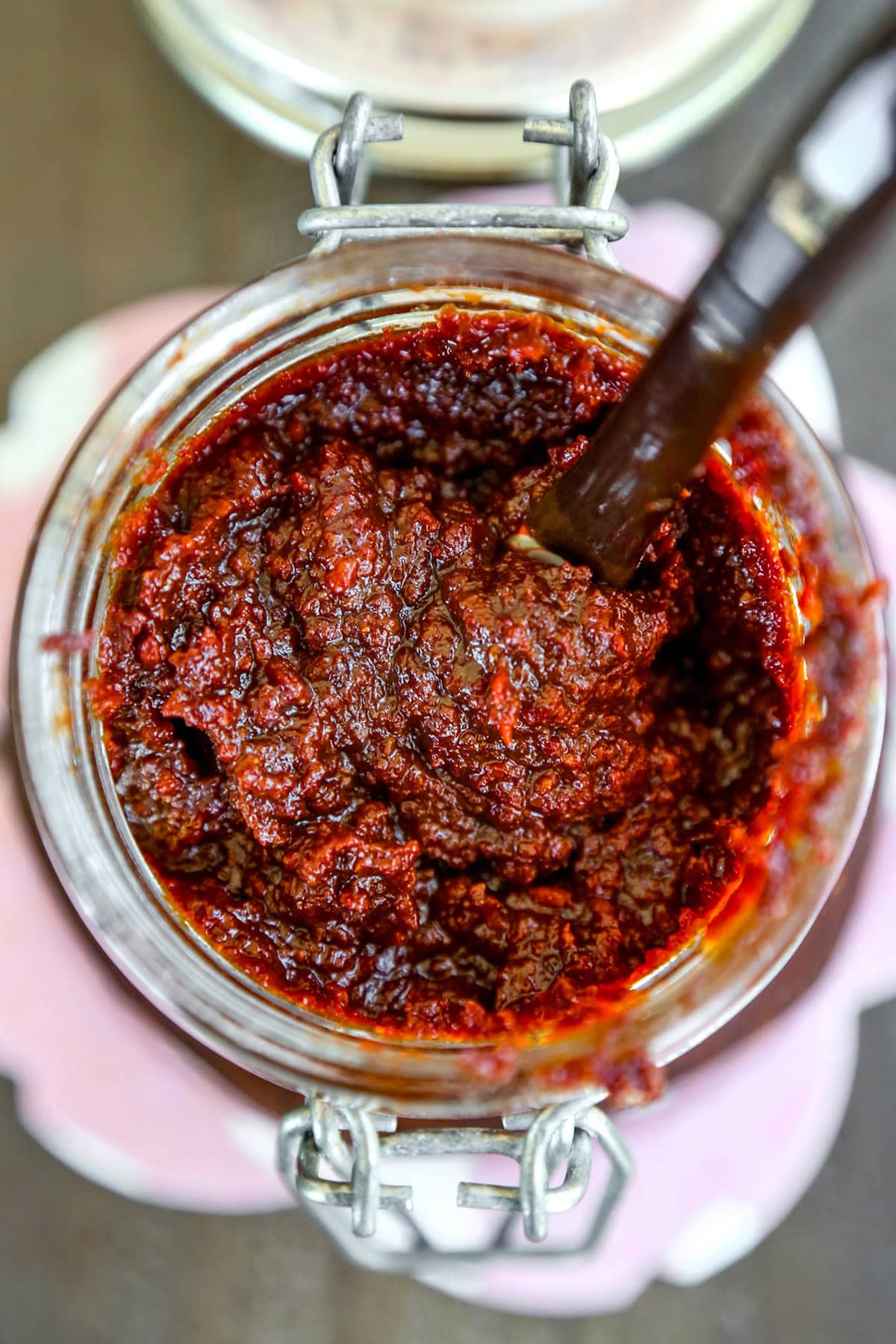The image depicts an open glass mason jar viewed from above, featuring a bright, seed-filled red jam that might be raspberry, blackberry, or boysenberry, though it could also be a seed-laden hot sauce. The jar, characterized by its metallic hooks on both the top and bottom, which are designed for securing the lid tightly, currently has the lid resting open. Inside the jar, a metallic handle of a spoon or fork is visible, dipping into the thick, reddish paste. The jar is situated on a pinkish floral doily, and the blurred background suggests it rests on a grayish-brown surface, possibly a wooden table. The overall setting and objects around the jar are out of focus, highlighting the textured contents within.